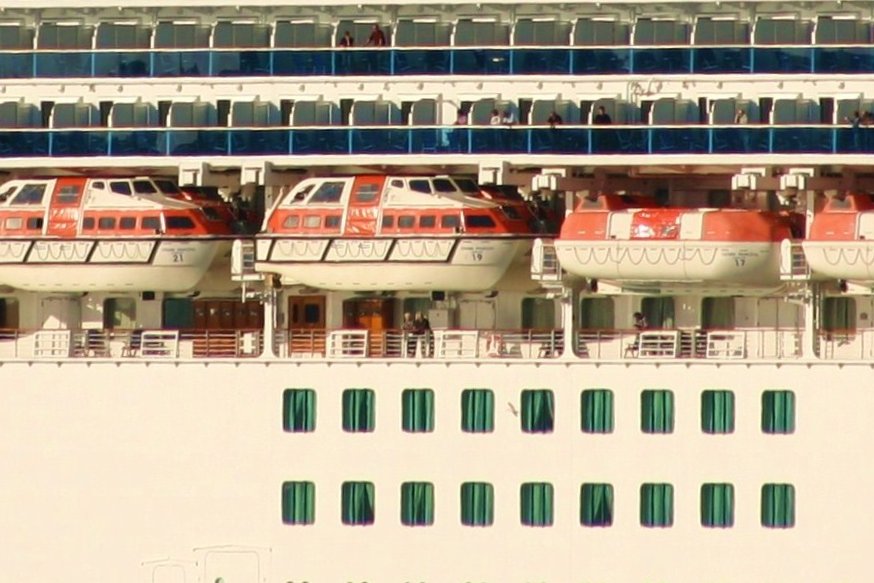This image depicts the side of an expansive cruise ship, showcasing multiple levels and various features. At the very top, there are two white tiers serving as balconies attached to passenger cabins. These balconies have barriers between each section, and several people can be seen standing in these spaces. The railings on the balconies feature blue window linings underneath.

Just below these balconies are emergency escape boats, identifiable by their orange and white color scheme, with white hulls and red sides, resembling lifesaver boats. Four such boats are clearly visible.

Below the escape boats, there is another deck featuring balconies with brown doors behind white railings. A couple of people can be seen on this balcony area, with one person notably leaning over the side railing.

At the bottom of the image, the ship's side shows two rows of windows, each adorned with green curtains. The area between the windows is a smooth, white wall, adding to the overall clean and structured appearance of the cruise ship.